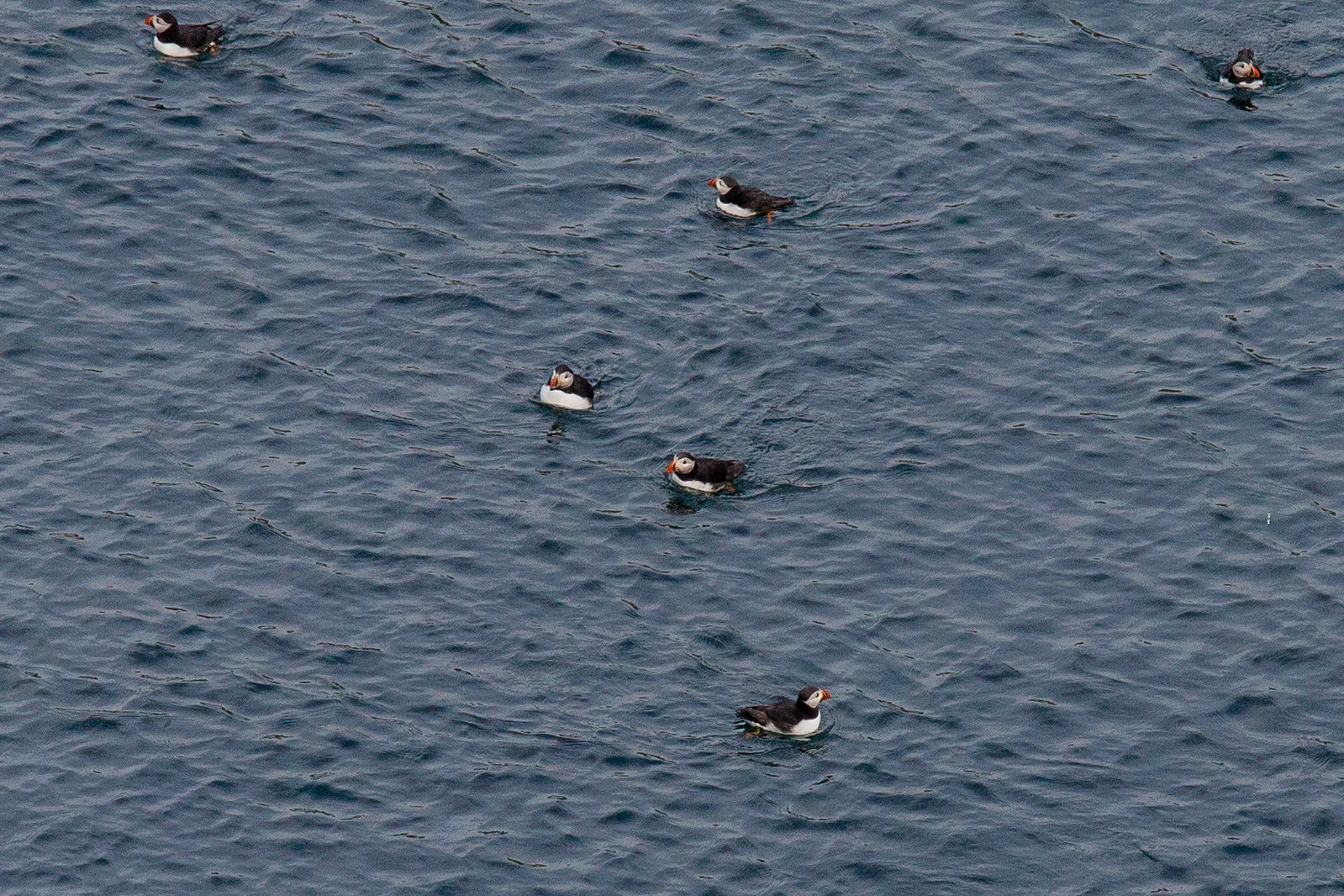This is a daytime color photograph showcasing a group of six puffins in a moderately wavy, deep blue-gray body of water. The puffins, identified by their striking black backs, white faces, white bellies, and bright orange beaks, are irregularly spaced and facing various directions. One puffin in the middle of the image, seen in a side profile facing left, floats serenely, while another nearby to the left offers a front view. Three puffins linger in the upper half of the image, with one each positioned at the top left, top right, and top center. A final puffin at the bottom center appears to be swimming with slightly open wings, giving a glimpse of its orange feet beneath the water. The gentle waves and light reflections add a sense of movement to the peaceful scene.